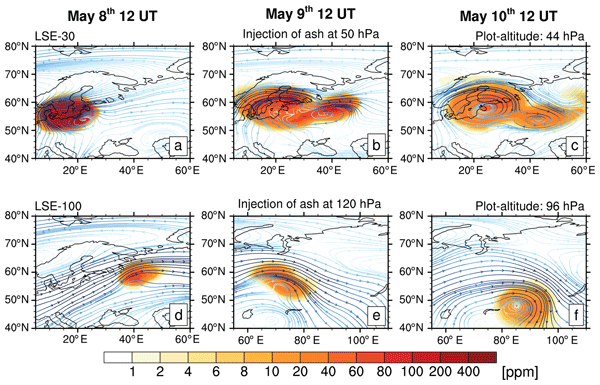The image features a detailed meteorological chart laid out in a 3x2 grid displaying six different visuals, each corresponding to specific dates and times: May 8th, 12 UT through May 10th, 12 UT. Each subplot is a degree map illustrating temperature variations using a range of colors—primarily reds, yellows, and oranges—indicating areas of heat concentration. The left axis of each subplot is labeled from 40 to 80 degrees, while the bottom axis shows coordinates from 20 degrees east to 60 degrees east. The chart also details conditions before and after the injection of ash at 50 HPA, with plot altitudes ranging between 44 and 96 HPA. The visuals effectively depict meteorologic changes over the selected period, likely tied to volcanic activity, as indicated by an LSE 30 injection.